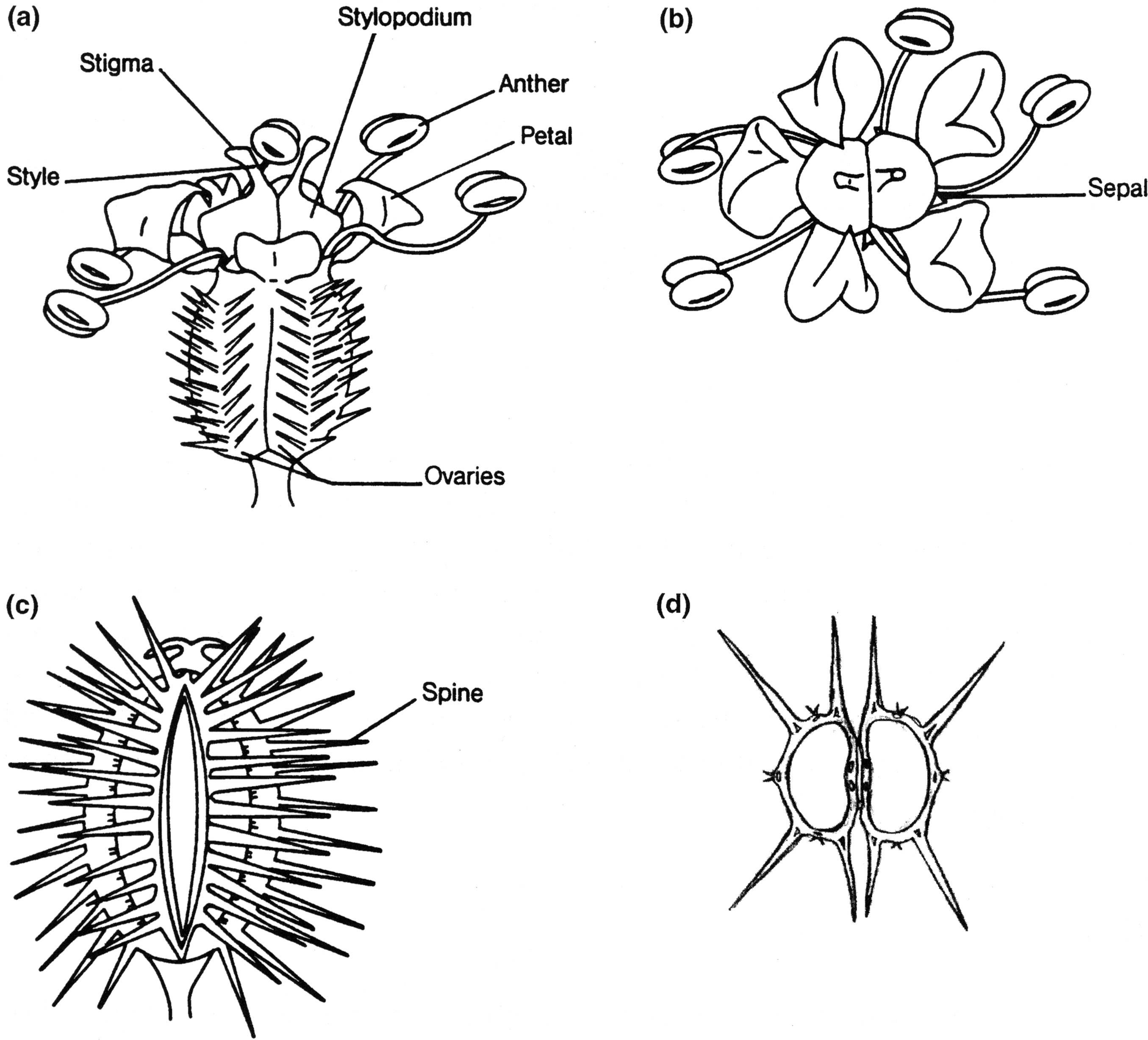This black-and-white scientific line drawing features four distinct images labeled A, B, C, and D. Each image illustrates a different part of a flower, meticulously detailed and labeled, reminiscent of diagrams found in science textbooks or journals. Image A is a comprehensive depiction of a fully labeled flower, detailing the stigma, style, stylopodium, anther, petal, and ovaries. Image B presents a close-up of a blooming flower's sepal. Image C focuses on a cross-section of a flower spine, while Image D illustrates a Venus flytrap, highlighting the mechanisms by which its teeth close around insects. The precise black labels are small and methodically placed, suggesting an educational purpose, possibly as a quiz answer key. All objects have a scientific aesthetic, emphasizing intricate floral anatomy.